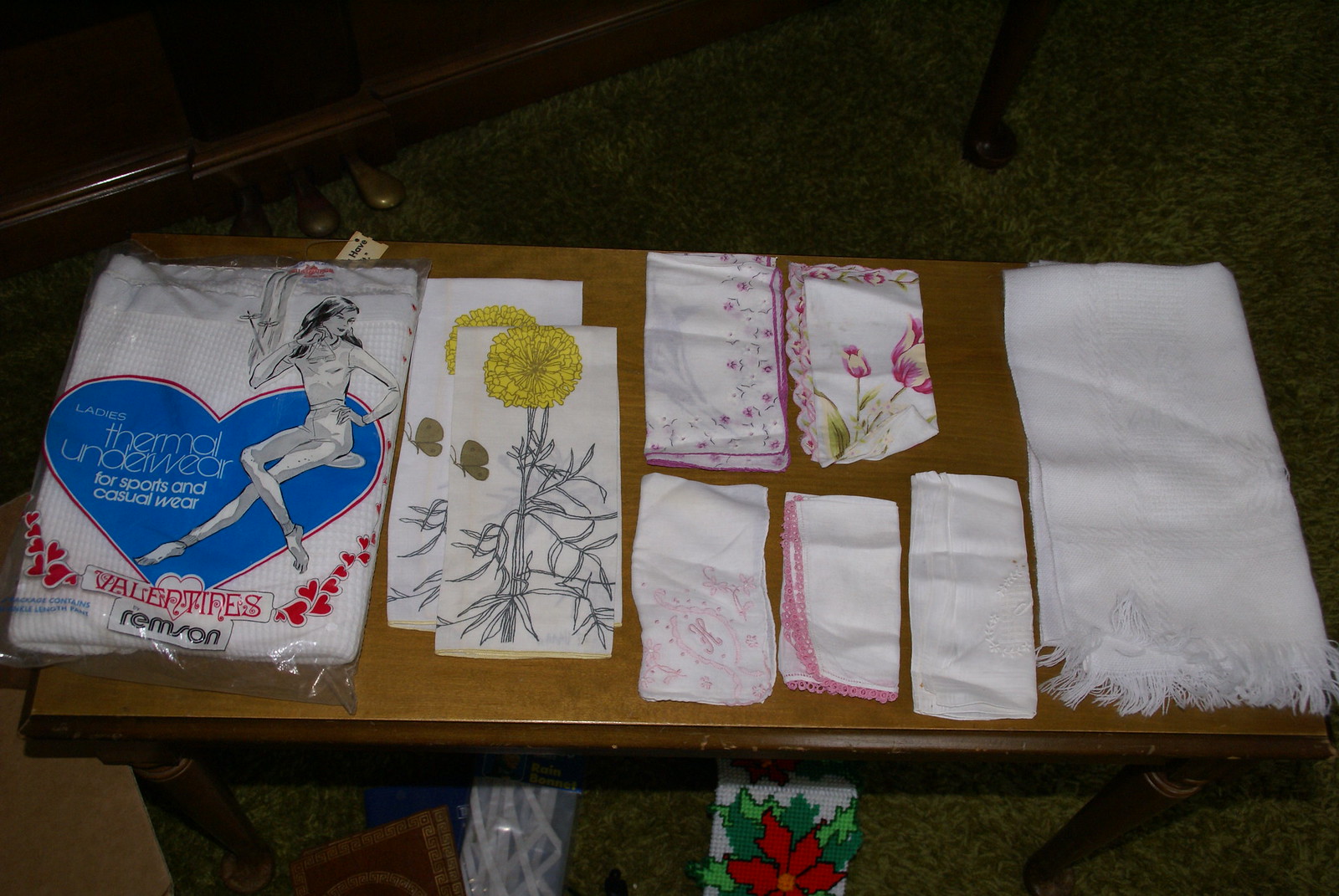The photograph features a small brown wooden side table, likely in a hallway, covered with an assortment of cloth items. Central to the arrangement is a package of women's thermal underwear adorned with a large blue heart and numerous small red hearts, promoting its use for sports and casual wear. The package prominently features an image of a woman sitting with her legs crossed and includes the word "Valentine's" in red. Surrounding this package are various folded cloth items. To the left, two handkerchiefs or small towels feature bright yellow flowers, possibly chrysanthemums, and black line drawings of stems and leaves. Adjacent to these are five smaller napkin-like cloths with pink embroidery. On the right side of the table, a larger white cloth, resembling a towel or tablecloth, is folded neatly with visible fringe at the ends. The background reveals a section of a dark wooden piano stool with three pedals, hinting at the photograph's setting, and a somewhat dirty green carpet beneath the table. The detailed curation of items suggests a deliberate decorative or thematic arrangement.